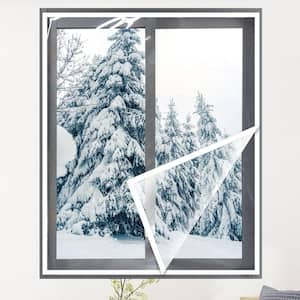The image depicts a window with a gray frame and a vertical gray strip running down its center. The window is set in a cream-colored wall. Outside, a snowy landscape features dark blue-gray evergreen trees heavily coated in snow, resembling a classic winter or Christmassy scene. The sky outside appears pure white, adding to the cold ambiance. A transparent plastic sheet, likely meant for insulation, covers the window, with its bottom right corner partially peeled away, revealing a crinkled reflection in the top left corner. The plastic film gives an impression of being either magnetically or velcro-attached to the window frame.